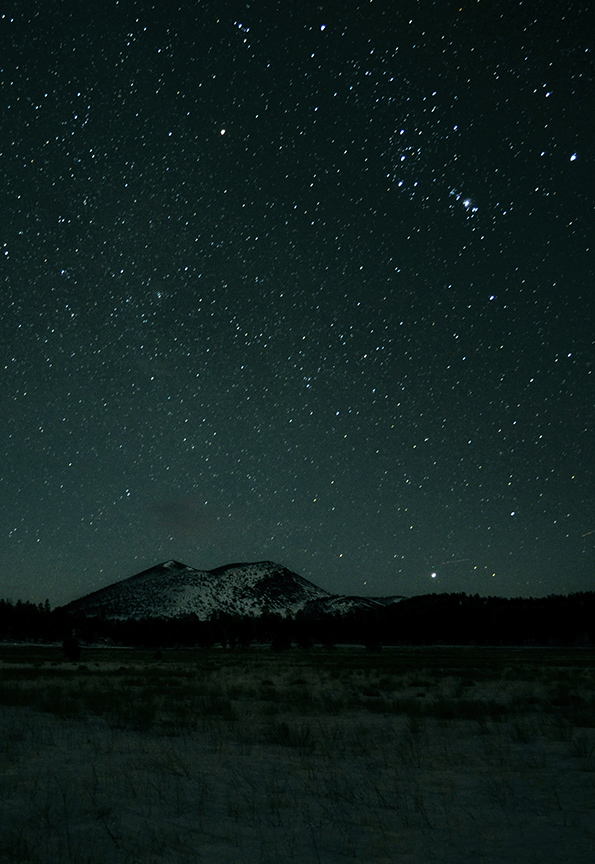In this captivating nighttime image, an expansive, sandy terrain stretches out darkly and sparsely from the camera's perspective towards a distant, formidable mountain. The foreground is mostly barren, dotted occasionally with scraggly plants, underscoring the land's inhospitable nature. Further away, a faint silhouette of trees hints at a small forest nestled at the mountain’s base. The mountain itself, with its twin peaks and gentle inclines dusted with snow, looms large under a star-studded sky. The scene is bathed in a grayish tint from the moonlight which softly illuminates the landscape. On the horizon, a subtle glow suggests the presence of a town or village beyond the mountain. The sky, transitioning from a lighter hue near the land to a deep black as it ascends, is densely packed with twinkling stars of white, orange, and yellow, creating a mesmerizing constellation display.